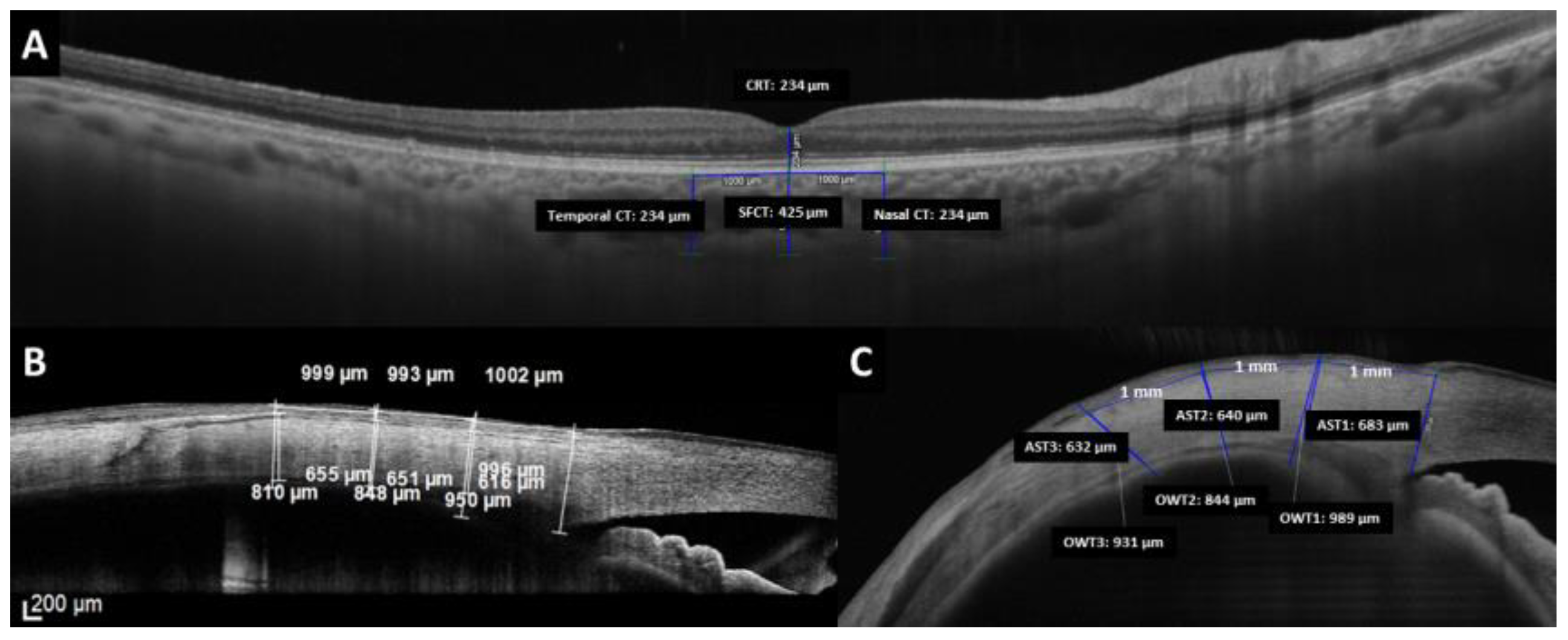This black-and-white image, possibly a scientific scan such as an x-ray or an electron microscope image, is horizontally oriented with intricate details. The background is black, while the scan itself displays varying shades of white and gray. Lettered segments, A at the top, and B and C in the lower sections, denote different parts of the scan. Blue lines are visible, indicating specific measurements. 

The image includes several measurements in micrometers, with text boxes displaying values such as "200 micrometers," "234 micrometers," "424 micrometers," "99 micrometers," "993 micrometers," and "1002 micrometers." The labels correspond to specific regions of the scan, mentioning terms like CRT, temporal CT, SFCT, and nasal CT.

While the precise nature of the scanned objects is unclear, they appear animal-like, with some segments resembling teeth. The top section might depict a part akin to the body of an organism. Despite the absence of identifiable eyes, the image offers a structured view, presenting a detailed, yet ambiguous, scientific depiction.